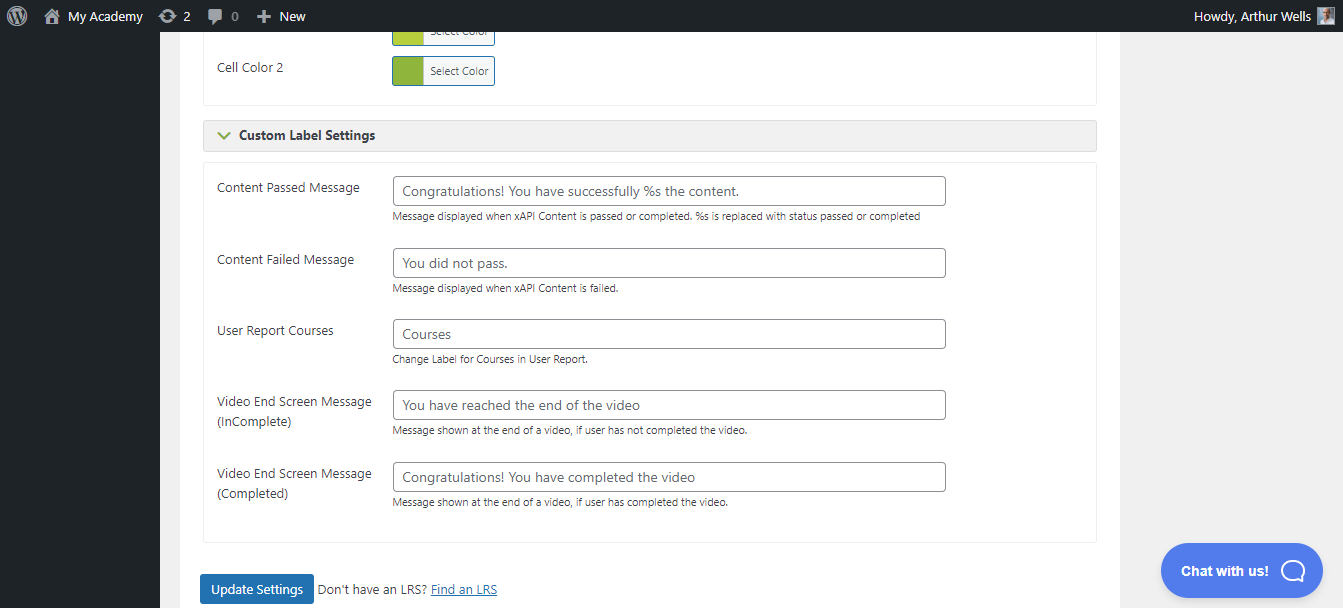The image features a predominantly gray background with several elements highlighted in contrasting colors. At the center, there is a gray circle with a black "W" in the middle, which appears to be a logo. Below it is the text "my academy" also in gray. 

To the right, there's a green square adjacent to a gray rectangle. Inside the gray rectangle, there are options including "Select Color," and "Custom Label Settings" displayed in black text.

Further down, a gray rectangle displays a couple of alert messages: one congratulating the user on successfully achieving something with the text "Congratulations! You have successfully [percent sign] s," and another indicating failure with the message "Content failed: You did not pass."

The user interface also includes various navigational and informational options like "User Report," "Courses," and "Courses Video and Screen Message." There is a video status message within parentheses, stating either "(Incomplete) You have reached the end of the video," or "(Completed) Congratulations! You have completed the video."

Finally, at the bottom of the image, there is a prominent blue oval button with the text "Chat with Us" written in white.